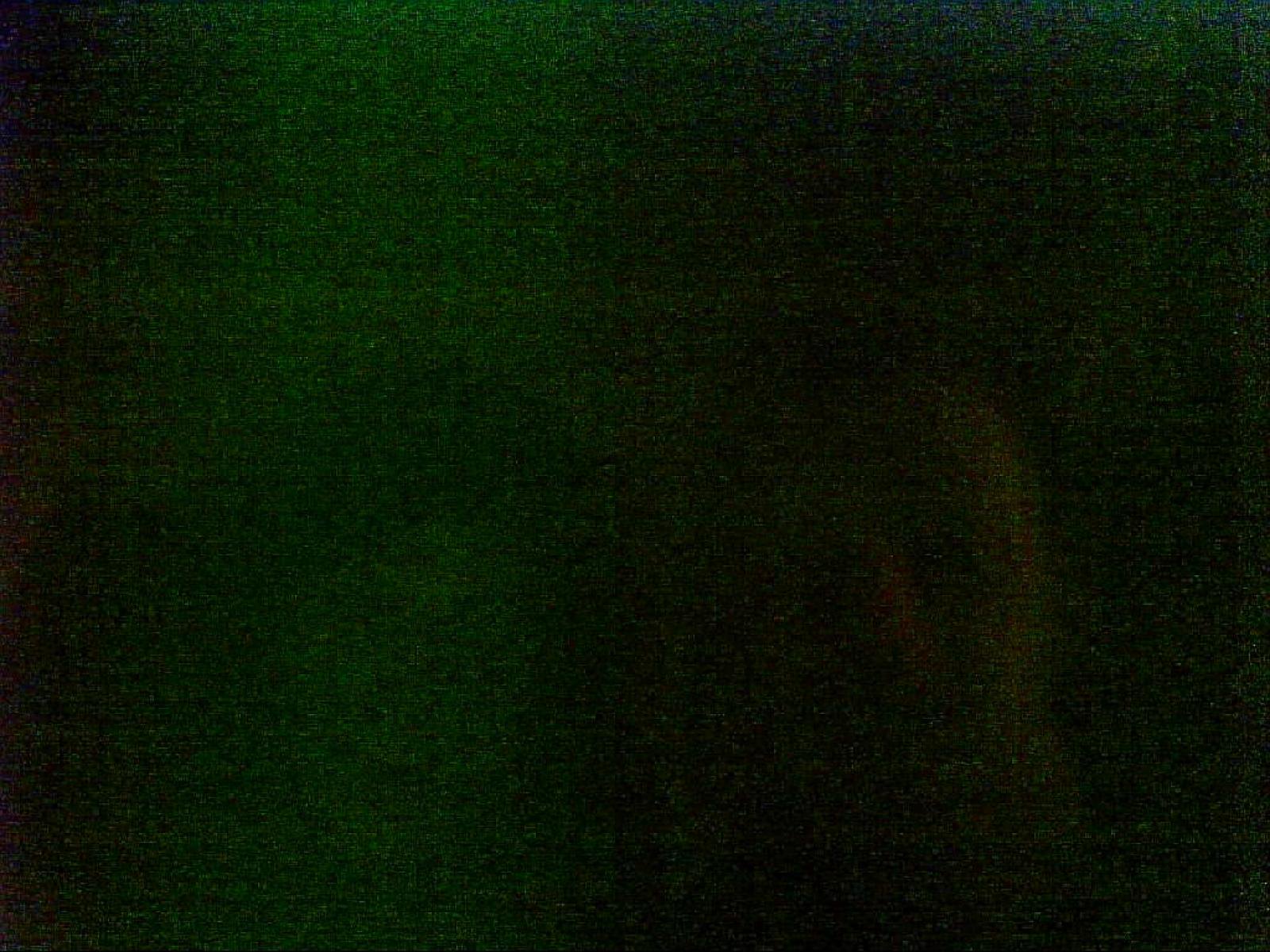The image is an extremely dark and blurry photograph dominated by black and green hues. The grainy texture suggests it may have been taken with a low-quality camera, possibly from the early 2000s without adequate lighting or a flash. The left side of the image primarily consists of dark shades with some very dark green near the top. Towards the right side, where the colors shift slightly, there appears to be an indistinct shape that could be interpreted as a person's face, with the nose and side profile faintly visible. Overall, the image's lack of clarity and detail makes it challenging to discern any specific elements beyond its grainy green and black composition.